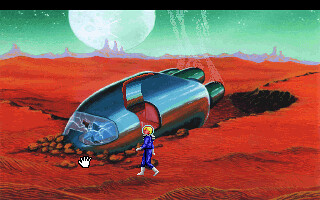A small rectangular image portrays a crashed silver spaceship on a desolate red planet. The spacecraft is angled, with its front end facing the bottom left and the rear end pointing towards the top right. A pronounced crater lies behind the spaceship, while dirt and rocks are heaped over its nose. The windshield is visibly cracked, and the side door hangs open. In front of the spacecraft, a lone astronaut is walking. The background features rugged, red, pointy formations stretching into the distance. The sky has an unusual green hue, dominated by a large, glowing bluish-green moon near the center.